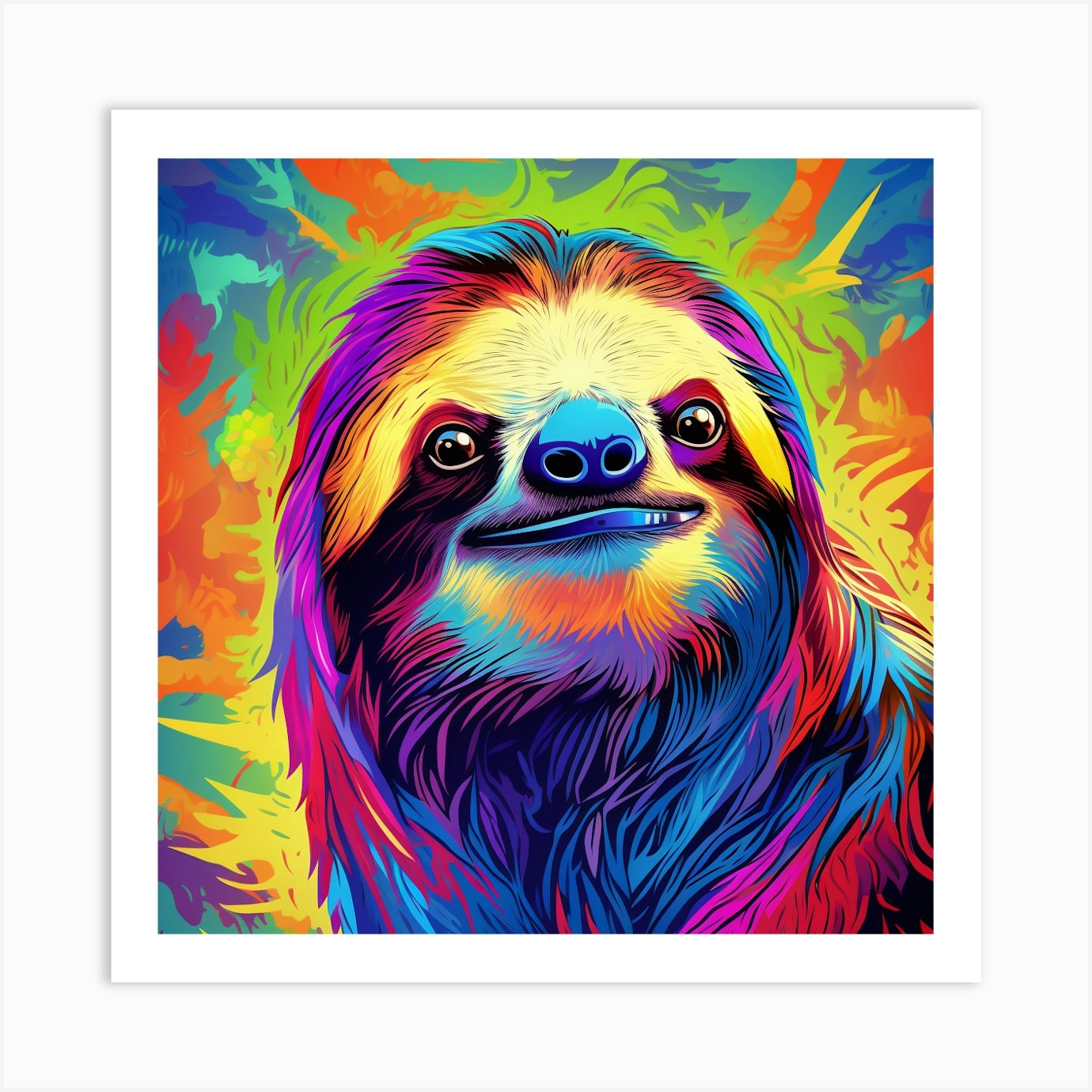The image is a vividly colored, modern rendition painting of a sloth, framed in white. The animal's face dominates the canvas, drawing immediate attention with its striking, bold colors and intricate details—a nod to pop art and psychedelic styles. The sloth's face has a yellow hue above its eyes on the forehead, while the area around its eyes is decked in purplish-red fur. Its eyes are a deep brown with black pupils, and the nose and lower lip are a striking blue, accented with black nostrils. The sloth's fur flaunts a vibrant array of colors, including blue, pink, purple, orange, and yellow, creating a mesmerizing multicolored tapestry. Its hair is symmetrically parted in the middle, giving it an almost styled appearance. The background features a captivating mix of lighter, brighter colors—lime green, yellow, orange, and various shades of blue—forming patterns that resemble leaves and trees, enhancing the overall psychedelic atmosphere. Flame-like motifs in the background add to the dynamism of the painting, making it both striking and fun.